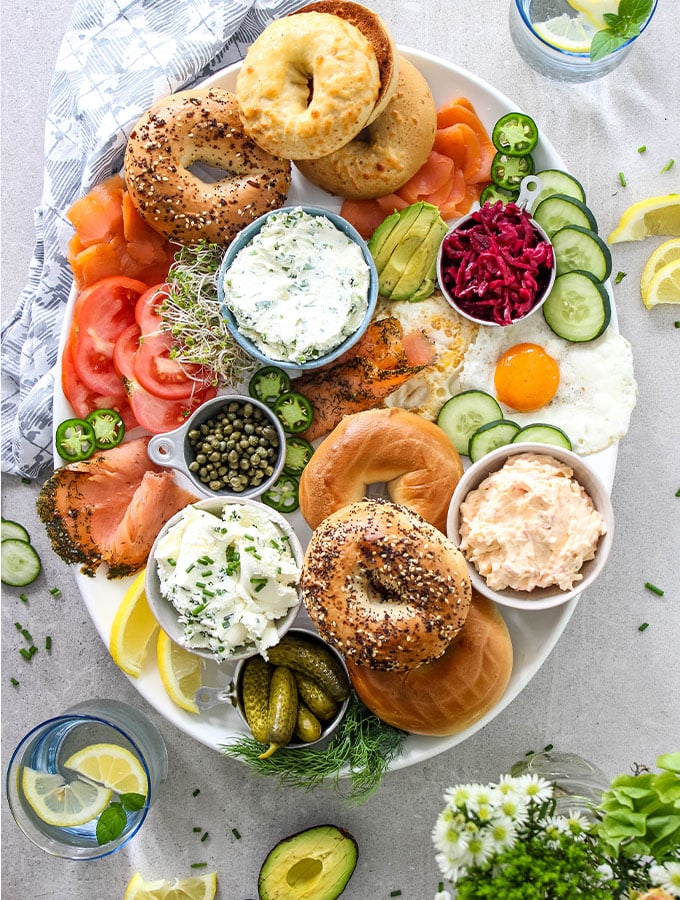This detailed photograph features a plentiful breakfast platter, predominantly showcasing an assortment of bagels that have been cut in half and toasted to golden perfection. Arranged on a large serving plate, the bagels are surrounded by a vibrant variety of fresh, sliced vegetables including tomatoes, cucumbers, pickles, and avocado halves. There are colorful bell peppers and zesty jalapenos adding a touch of heat. A generous helping of smoked salmon and several cups containing a trio of dips, likely various flavors of cream cheese such as one with chives or lox, enhance the platter’s appeal. Capers are dotted across the arrangement, perfect for garnishing the bagels.

This inviting spread rests on a white tablecloth-covered table, alongside several glasses of water adorned with refreshing lemon slices. Nestled among the food, a small cup of dill pickles and a bunched-up napkin with a blue and gray design are visible. Additionally, a small flower arrangement provides a hint of elegance and color to the setting, perfect for an enjoyable and hearty breakfast experience.